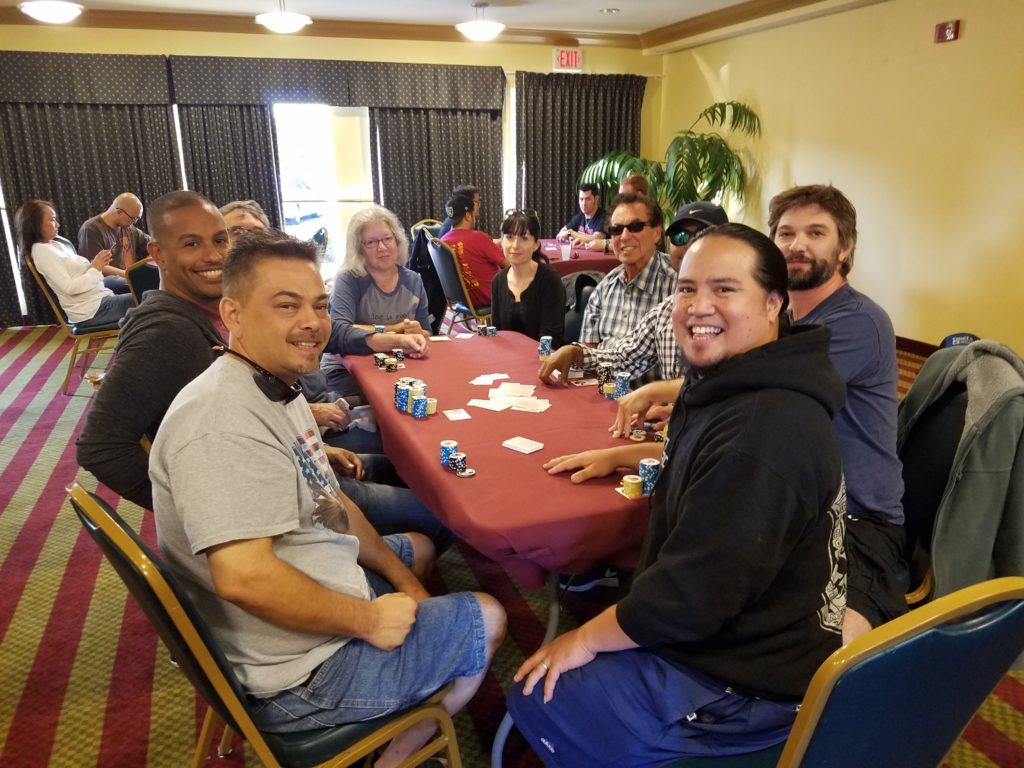A photograph captures an indoor scene where a group of people are engaged in a lively poker game. The room features a window on the far side, adorned with dark gray curtains that are mostly drawn closed, except for a small gap in the center. Suspended from the ceiling in this gap are three light fixtures that illuminate the room. Above the window on the opposite wall, an exit sign glows, with an artificial plant positioned on the floor beneath it. In the background, two additional tables are visible. The focal point of the image is a rectangular table directly in front of the camera, around which nine or ten people are seated on chairs with dark blue backs and seat cushions supported by metal legs. The players have turned around in their seats to smile at the camera, their expressions radiating warmth and camaraderie. The table is scattered with poker chips and playing cards, indicating they are immersed in a game.